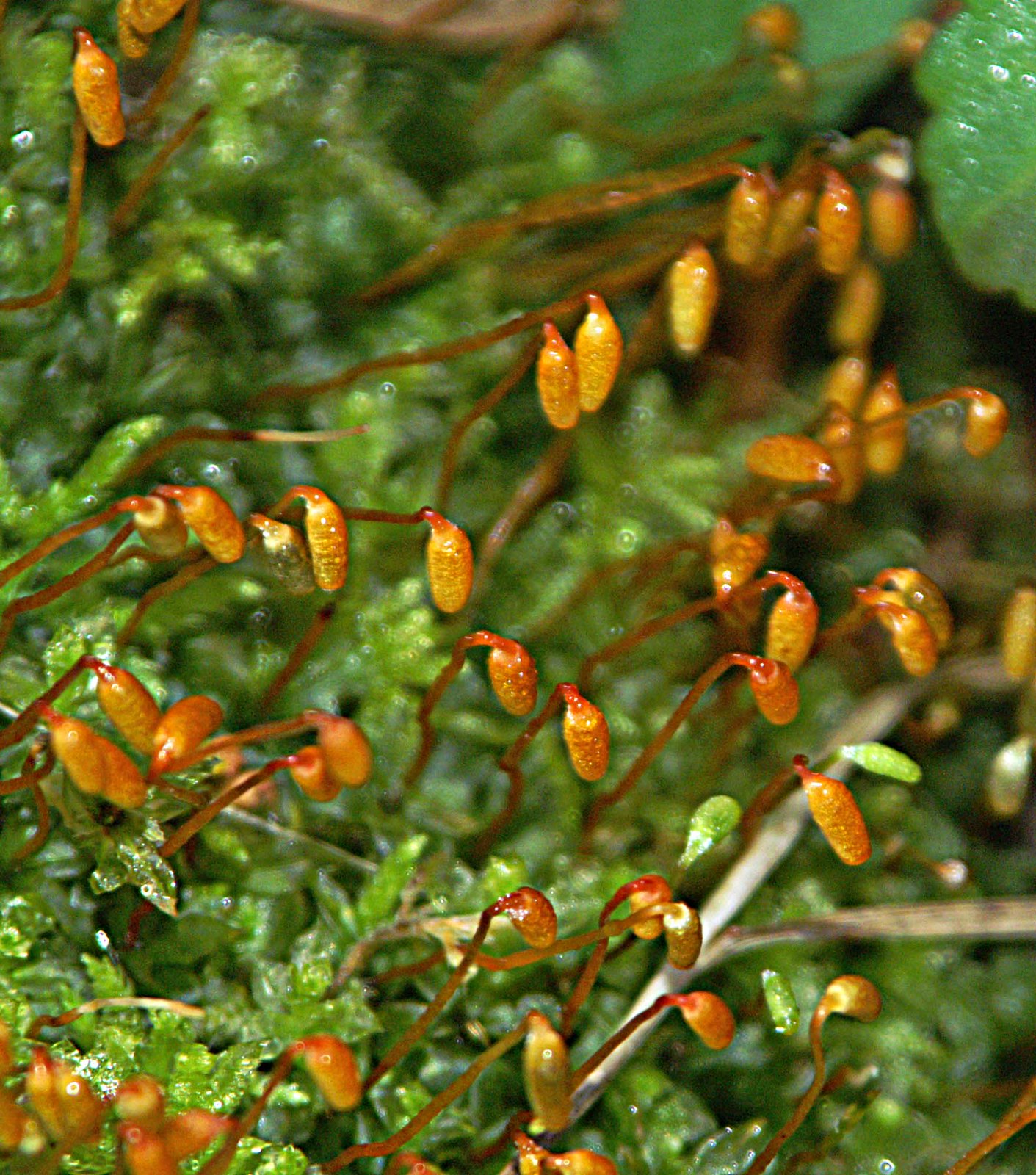This photograph captures an up-close view of a cluster of small, emerging plant buds. The main focal point is a vine-like structure with its brown shoot adorned with oval-shaped pods that are a vibrant orange or yellowish-orange color. These intriguing buds, resembling trichome-like antennas, give a dynamic sense to the plant. The background reveals a lush forest green mossy substrate, indicating a possible moist, outdoor environment enhancing the texture and depth of the image. Scattered across the scene are about 25 to 30 of these tiny sprouting buds, each approximately an inch tall, giving the appearance of new life emerging and uniformly leaning to the right, adding a palpable sense of growth and direction to the composition.